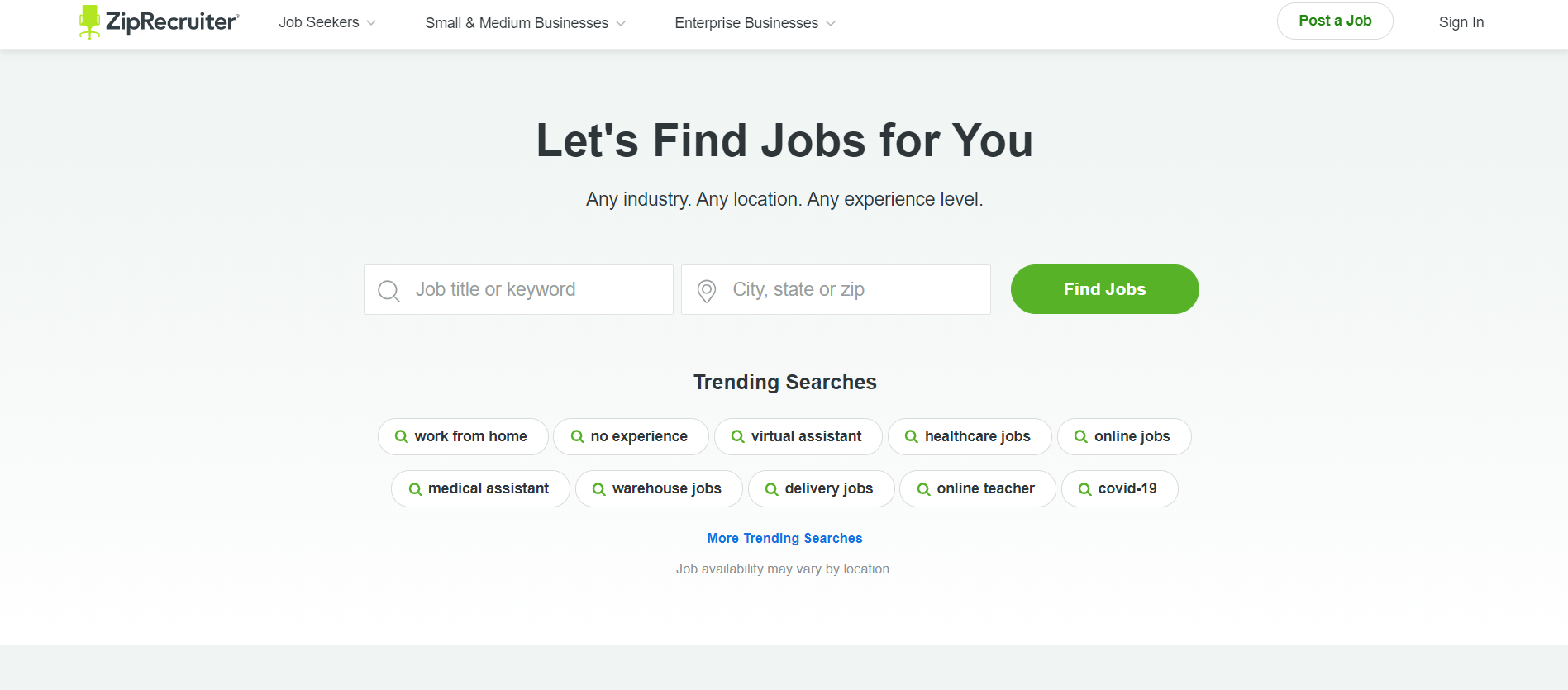The top of the image prominently features the "ZipRecruiter" logo on the left side, accompanied by an icon resembling a green chair. To the right of the logo, there are navigational options labeled "Job Seekers," "Small and Medium Businesses," and "Enterprise Businesses." A bold button labeled "Post a Job" is situated nearby. Towards the upper-right corner, there's an option for users to "Sign In."

Beneath this header, a gray section dominates the middle of the image, showcasing large, bold black text that declares, "Let's Find Jobs For You." Directly below this, a tagline reads, "Any Industry, Any Location, Any Experience Level."

Further down, there are two input boxes: one with a magnifying glass icon labeled "Job Title or Keyword," and another with a location pin icon labeled "City, State or Zip." A prominent green button labeled "Find Jobs" invites users to initiate their search.

At the bottom of the image, under the heading "Trending Searches," there are ten buttons, each featuring a magnifying glass icon. The buttons are organized from top left to bottom right, and are labeled as follows: "Work From Home," "No Experience," "Virtual Assistant," "Healthcare Jobs," "Online Jobs," "Medical Assistant," "Warehouse Jobs," "Delivery Jobs," "Online Teacher," and "COVID-19."